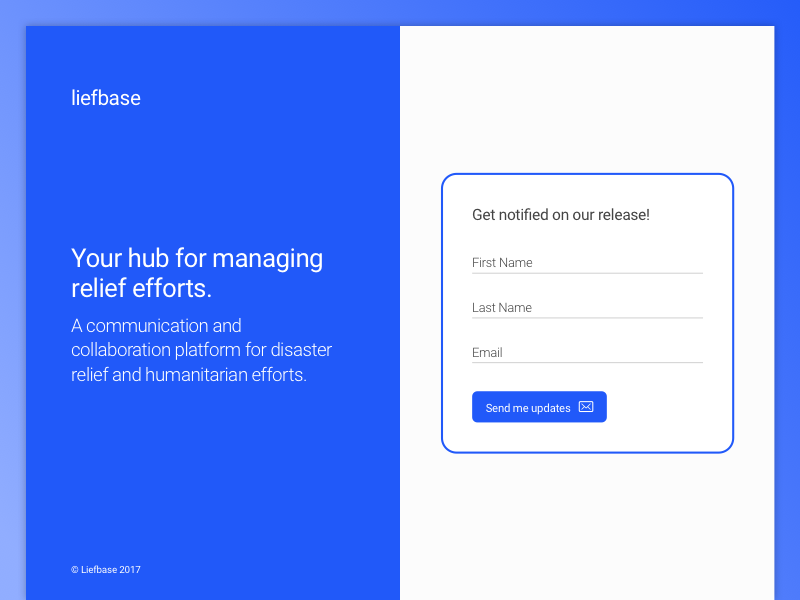The image portrays a user interface designed for managing disaster relief efforts on a platform branded as "Leaf Base." The interface features a registration section where users can sign up to receive updates about relief efforts. Users are prompted to enter their first and last names and then click a "Send Me Updates" button. The background of the interface is a soothing blue, creating a calm and professional ambiance. Prominent text conveys that Leaf Base is a communication and collaboration platform dedicated to disaster relief and humanitarian work, emphasizing its role as a hub for coordinating and disseminating critical information during emergencies.